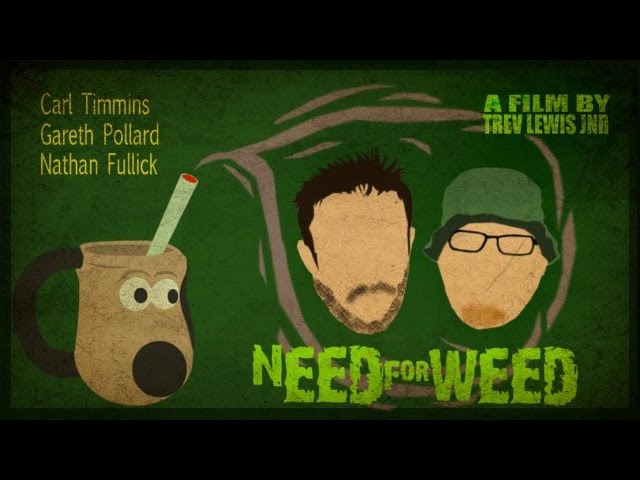This poster for the film "Need for Weed" features a dark green background framed by black banners at the top and bottom. On the top left, in yellow text, are the names: Carl Timmons, Gareth Pollard, and Nathan Fulick. Below these names is a coffee mug shaped like a dog's head, tan in color with white eyes and a large brown nose, and a black handle resembling the dog's ear. From the mug, a lit joint or blunt emits swirling smoke, leading to two faceless, floating heads. The head on the left has dark, short, spiky hair, a mustache, and a light beard, while the head on the right wears narrow-rimmed glasses and a green bucket hat with a goatee shadow. At the top right, green text reads, "A Film by Trev Lewis JNR." Prominently at the bottom, the film’s title "Need for Weed" is displayed in bold, bright green letters.